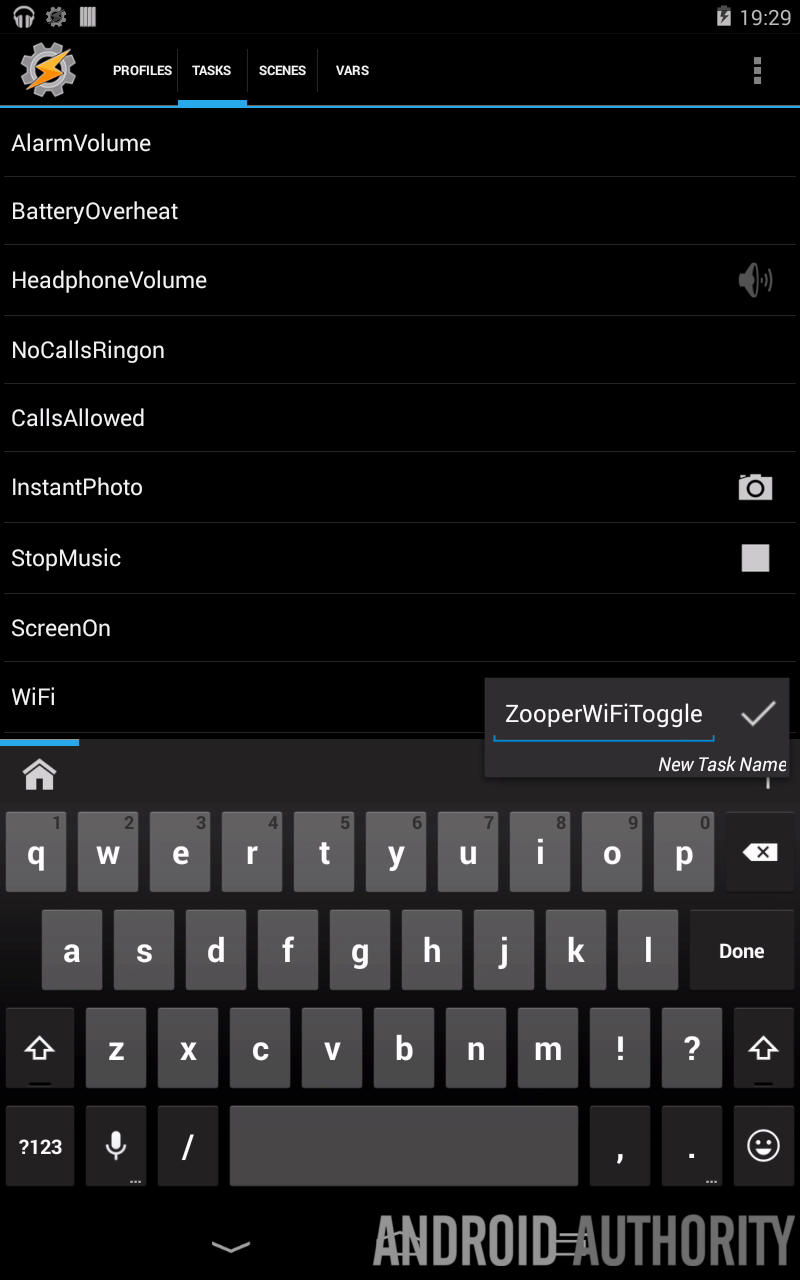This image is a screenshot from a mobile application described on a webpage by Android Authority, captured at 7:29. At the top of the screen, there's a gray circular icon with an orange lightning bolt through it, indicating the active page, which is the "Tasks" tab of the app. The interface displays a list of tasks including "Alarm Volume," "Battery Overheat," "Headphone Volume," "No Calls," "Ring on Calls," "Allowed Instant Photo," "Stop Music," "Screen On," and "Wi-Fi." 

Each task has various icons next to it, representing their functions. "Headphone Volume" features a gray microphone icon emitting sound waves, indicating it controls the headphone volume levels. "Allowed Instant Photo" is accompanied by a gray camera icon, suggesting functionality for immediate photo capture. "Stop Music" has a gray and white square box, likely indicating a command to halt media playback. "Wi-Fi" includes a reference to "Zooper Wi-Fi toggle," suggesting integration with the Zooper widget for toggling Wi-Fi status.

Below this list, there is a section labeled "New Task Name," followed by a QWERTY keyboard displayed on the phone, ready for input. The overall design of the app is utilitarian, focused on task management and automation, as evidenced by the detailed icons and task labels.